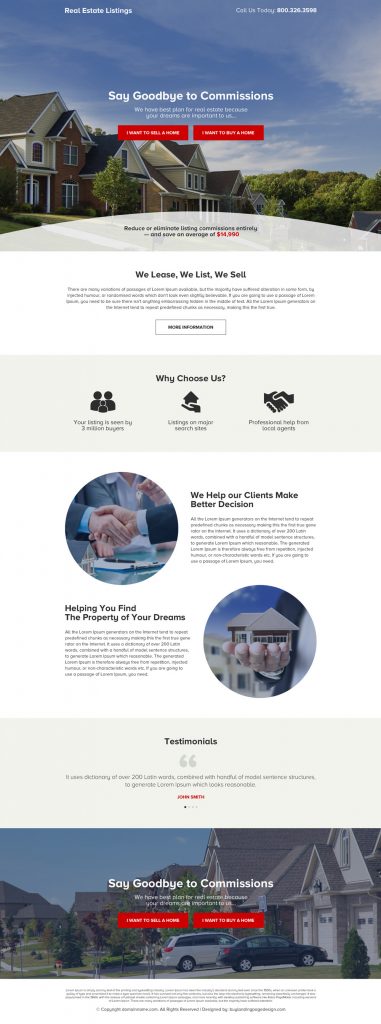The webpage screenshot for the real estate listings website features a well-organized layout designed to capture user interest and provide crucial information efficiently.

At the top left-hand corner, the website prominently displays "Real Estate Listings" in white. On the right-hand side, there's a call-to-action encouraging visitors to "Call Us Today," accompanied by a telephone number. This header is set against a vibrant background showcasing various houses under a clear blue sky.

Centrally positioned on the page, in bold white lettering, is the headline "Say Goodbye to Commissions," emphasizing a key selling point of the service. Beneath this, there are two small-font red buttons intended for further interactions.

Below this section, a white panel introduces a succinct message with a black heading that reads "We Lease, We List, We Sell." Following a brief paragraph of explanatory text, there's a white button designed for immediate action.

Moving further down, a grey panel presents a compelling case for the service with the heading "Why Choose Us?" in black. This section features three icons, each highlighting a unique benefit of the firm's real estate services.

Below this grey panel is a large white section containing two illustrative circles. One circle shows a handshake, symbolizing agreement or deal-making, while the other features a row of houses. Accompanying these images are detailed texts and headings, aligned on opposite sides of the pictures to provide clear information.

Another grey panel follows with a simple yet powerful heading: "Testimonials." This section likely includes client reviews to build trust and credibility.

Finally, the page concludes with a visually cohesive panel, mirroring the initial header, reiterating "Say Goodbye to Commissions" with the same two red buttons, reinforcing the main value proposition of the website.